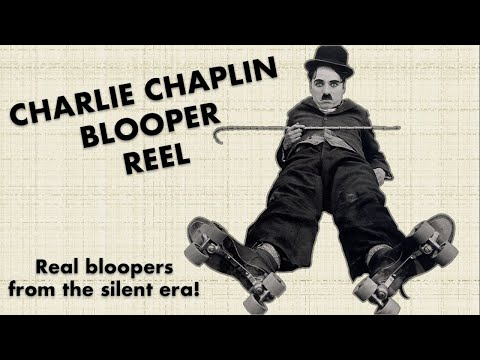The horizontally oriented image features a poster-style design with black bars on the top and bottom. Against a beige checkered canvas background, it prominently displays black text on the left side that reads "Charlie Chaplin Blooper Reel, real bloopers from the silent era." On the right, there is an edited photographic cut-out of Charlie Chaplin himself, providing a comical and exaggerated bottom-up perspective. Chaplin is dressed in a black top hat, black suit jacket, black pants, and gray shirt. He is clearly identifiable by his small, iconic black mustache and is holding a cane in his right hand. He is also wearing roller skates and his left hand is slipped into his pocket. Chaplin gazes directly at the camera with a wide-eyed expression, seemingly making eye contact with the viewer. His stance, enhanced by the low angle, makes his roller-skated feet and his overall figure appear slightly oversized and humorous. The black and white color scheme of the photograph contrasts with the textured background, creating a striking visual designed to evoke the slapstick charm of the silent film era.